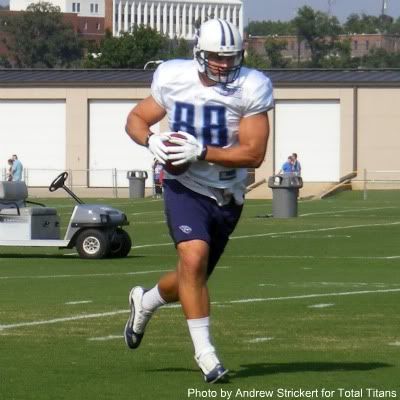In this detailed outdoor photograph, a professional football player, number 88, is captured mid-run across a vibrant green grass field. He is wearing a distinctive uniform featuring a white jersey with blue stripes and the number 88 prominently displayed. His head is protected by a white helmet with blue stripes down the center and a black face mask, while his hands, wearing white gloves, securely hold a football in front of his stomach on his left side. He sports blue shorts, white socks just past his ankles, and white and blue shoes.

The player appears to be twisting slightly as he runs towards the right side of the image. In the immediate background, there is a beige industrial-looking building with large white doors and a black roof. To the left, a golf cart is visible, and further back, you can observe another tall structure with white columns surrounded by lush greenery.

Overlaid on the photograph, towards the center, is the text "Photo Bucket" followed by "Protect More of Your Memories for Less" in a gray bar with green text. At the bottom right corner, a caption reads "Photo by Andrew Strickert for Total Titans," indicating the professional nature of the image and associating it with the Tennessee Titans football team.